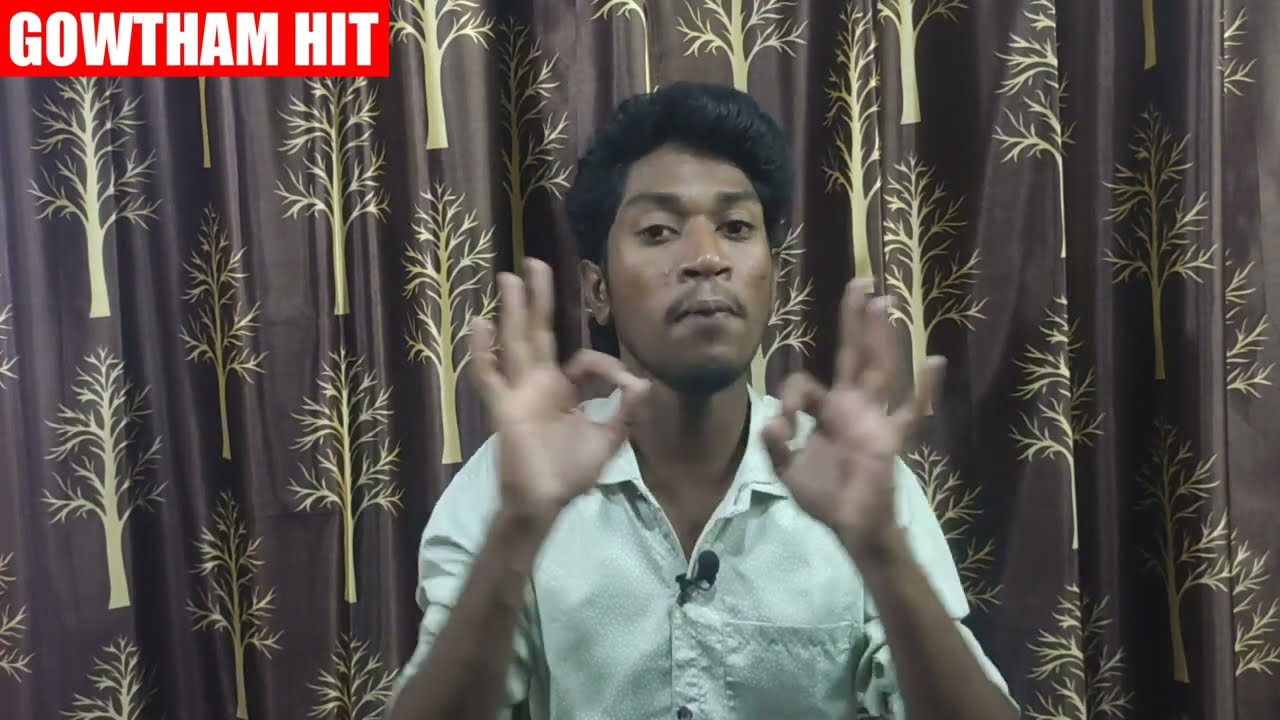A photorealistic image captures a South Asian man gesturing towards the camera with his hands forming the "okay" symbol, where his index fingers and thumbs are touching and the rest of his fingers are extended outward. He is centered in the image and is visible from his torso to the top of his head. The man has short, combed-back brown hair and is wearing a light sea green collared shirt with a pocket on the right side of his chest. A black microphone is clipped to his lapel. Behind him hangs a dark-colored curtain, which features a pattern of cartoonish yellow leafless trees. In the top left corner of the image, there is a red rectangular box with the text "Gautham Hit" written in white capital block letters.